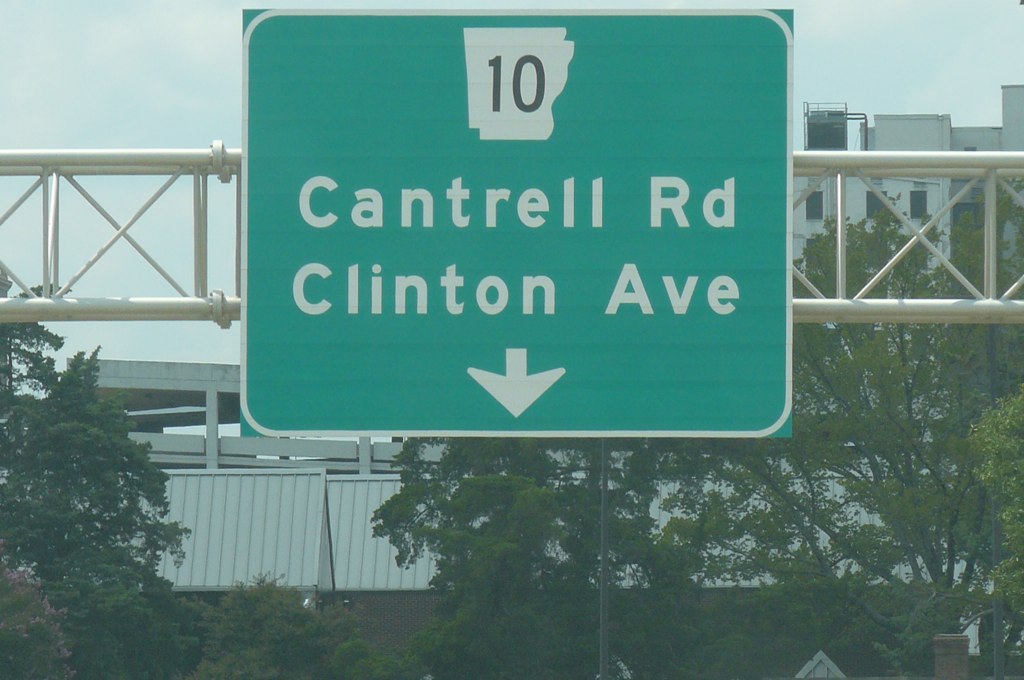The image depicts a clear, sunny day with light blue skies and scattered white clouds. Dominating the scene is a large, green overhead highway sign supported by a sturdy girder beam that spans the road. The sign prominently displays in white text the road number "10," along with the labels "Cantrell Road" and "Clinton Ave," accompanied by a downward-pointing arrow. Behind the sign, a long factory building with a white facade and visible air conditioning units on the roof stretches horizontally across the photo. In front of the factory, the tip of a house roof is visible, and the background is dotted with numerous green trees. Additionally, a white awning extends across most of the photo above the factory building. The setting is consistent with daytime, suggested by the bright light and lack of dense clouds.